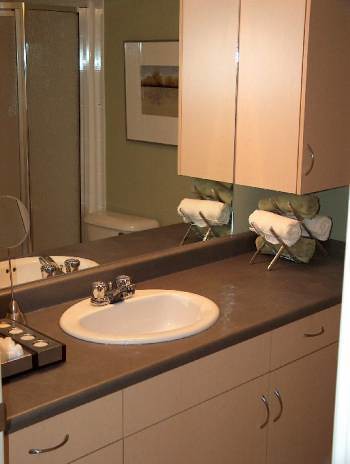This photograph captures an inviting and meticulously organized home bathroom. The centerpiece is a brown countertop featuring a pristine round white sink, complete with shiny faucets and knobs for hot and cold water. To the left of the sink, a small container, likely holding small candles, adds a touch of coziness. On the right side, a compact metal towel rack displays a neat arrangement of hand towels—two green and two white—rolled up perfectly. Above the counter, a light brown cabinet with a silver handle offers additional storage, complemented by the drawers and cabinets below. The large mirror behind the sink reflects the tranquil green walls adorned with a piece of artwork, enhancing the room's serene atmosphere.